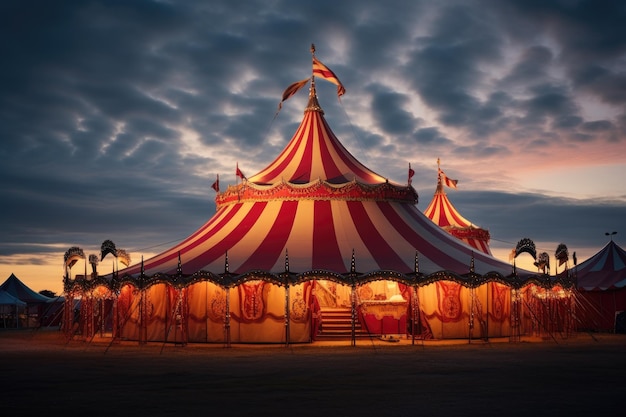Against a dramatic dusk sky filled with deep, dark clouds, an ornate circus tent stands prominently in an outdoor setting, exuding an air of nostalgic charm and vibrant allure. The grand circus tent is adorned with red and white stripes and topped with gold posts and red and white flags flapping gently in the breeze. The tent showcases multiple elaborate layers, with the middle section resembling a crown, accentuated by additional red flags. Ornate poles skirt the perimeter, firmly anchoring the structure into the ground. The entrance to the tent is invitingly lit by a warm, yellow glow, with steps leading up into the interior, partially veiled by draping white fabrics. In the backdrop to the right, a smaller, similarly striped tent echoes the majesty of its larger counterpart. The foreground remains shadowed, enhancing the illuminated elegance of the circus scene. The entire setup, bathed in the ethereal light of the setting sun, suggests an enchanting evening ahead, even as the dark clouds hint at a possible earlier rain.